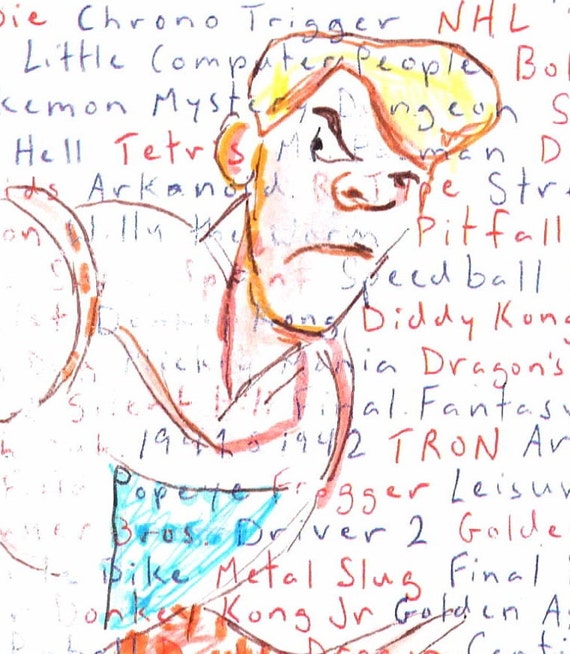The image is a hand-drawn illustration prominently featuring a male figure with distinctive blonde hair and a muscular build. The figure, outlined in orange and red, displays a blue shield on his chest and a skull-like face, complete with a frown, large eyes, and a prominent nose. The character’s hair is highlighted with yellow, adding a touch of color to the primarily blue and orange sketch. Surrounding and overlapping this figure are numerous words written in dark blue and red, some of which are partially erased. These words include names like Chronal Trigger, NHL, Little Computer People, Tetris, Arkanoid, Pitfall, Speedball, Tron, Frogger, Metal Slug, Leisure, and Kong, suggestive of various video games. The illustration appears as if it was created on a page already filled with text, contributing to the intricate and layered visual composition.